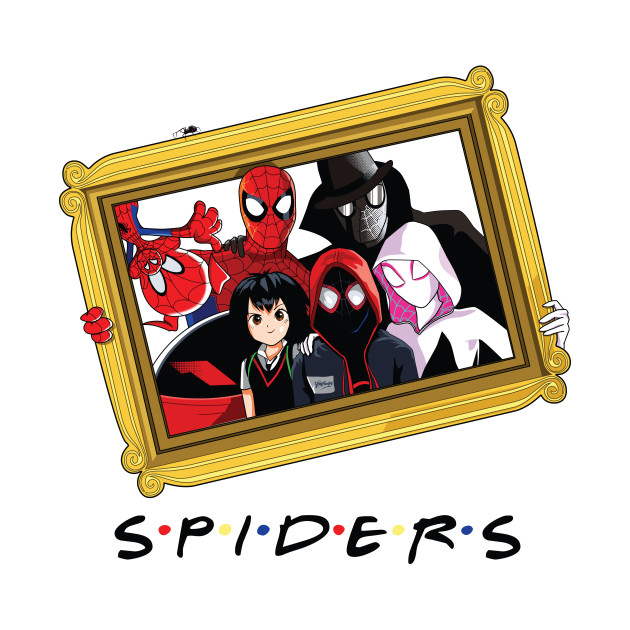The image is a completely digital illustration set against a white background. At the top of the image, slightly askew, is a gold, rectangular picture frame. A small black spider crawls on the top of the frame. Inside the frame, there are various cartoon characters all portrayed in a distinctive, animated style. In the top left corner of the frame, there is a "Porky the Pig" Spider-Man. In the middle top section, we see a standard Spider-Man. The top right section features a Spider-Man dressed in all black, wearing a trench coat and a hat. The bottom left corner of the frame displays a normal-looking girl with black hair and brown eyes. The center of the frame includes a dark, hooded Spider-Man with glowing red eyes, while the bottom right corner features a glowing-eyes female Spider-Woman dressed in pink. Beneath this framed artwork is the word "spiders" written in black cursive script, styled with colored dots—red, yellow, and blue—between the letters, resembling the 'Friends' TV show logo. The colors present in the image include black, yellow, gold, gray, white, pink, silver, red, and blue.